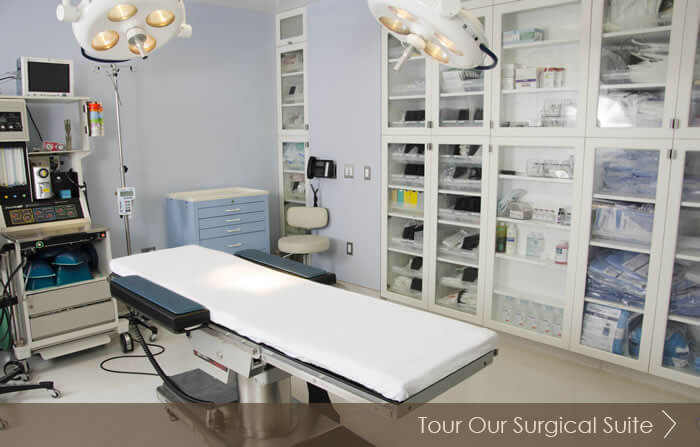The image depicts a well-equipped surgical suite or doctor's office. At the center of the room stands a large operating table with a white cover and dark blue armrests, mounted on a silver hydraulic mechanism that allows it to adjust in height and orientation. Above the table, two large surgical lights hang from the ceiling, each encased in circular frames with four bulbs. 

To the left of the bed, there is a movable desk with assorted clinical supplies, some of which are cyan in color, alongside small LCD screens and the legs of a wheeled chair peeking into the frame. On the right side, there is a mobile tray with multiple cyan-colored drawers next to a beige-cushioned rolling chair. An IV pole is situated at the head of the bed.

The back wall features large, see-through metal cabinets with many organized sections containing patient gowns, bottles of medicine, medical supplies, and monitoring devices. The walls of the room are painted cyan or gray, adding a clean and sterile ambiance. At the bottom of the image, a brown rectangle with white text reads "tour our surgical suite" accompanied by an arrow pointing to the right, suggesting that the photo was captured from a computer screen. Overall, the room is meticulously organized and equipped with state-of-the-art medical equipment.